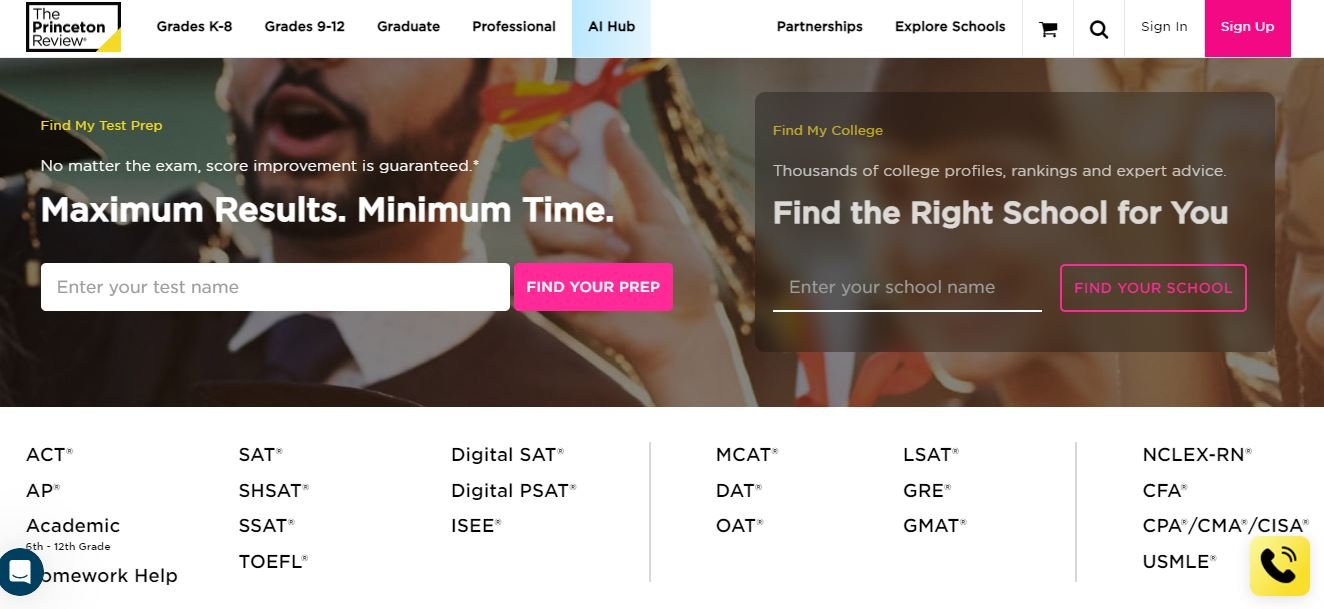The screenshot captures the homepage of The Princeton Review website. The website name, "The Princeton Review," is prominently displayed in the top left-hand corner. Adjacent to this, there is an off-white toolbar featuring various educational categories and options, including "Grades K-8," "Grades 9-12," "Graduate," "Professional," "AI Hub," "Partnership," "Explore Schools," "Cart," "Search," "Sign In," and "Sign Up."

Beneath the toolbar is a prominent rectangular image, approximately 8 by 3 inches in dimension, showcasing the lower part of a person's face and a hand. Superimposed over this image is a block of motivational text encouraging users to "Find my test prep," with assurances of score improvement and efficient results. The text further includes a search bar prompt, "Enter your test name," and additional options to find test preparation resources or college information.

The section following the image details various examinations and academic services provided by The Princeton Review, without a distinct heading. The extensive list of tests includes: ACT, AP, academic homework help, SAT, SSAT, SHSAT, TOEFL, Digital SAT, Digital PSAT, ISEE, MCAT, DAT, OAT, LSAT, GRE, GMAT, NCLEX-RN, CFA, CPA, CMA, CISA, and USMLE.